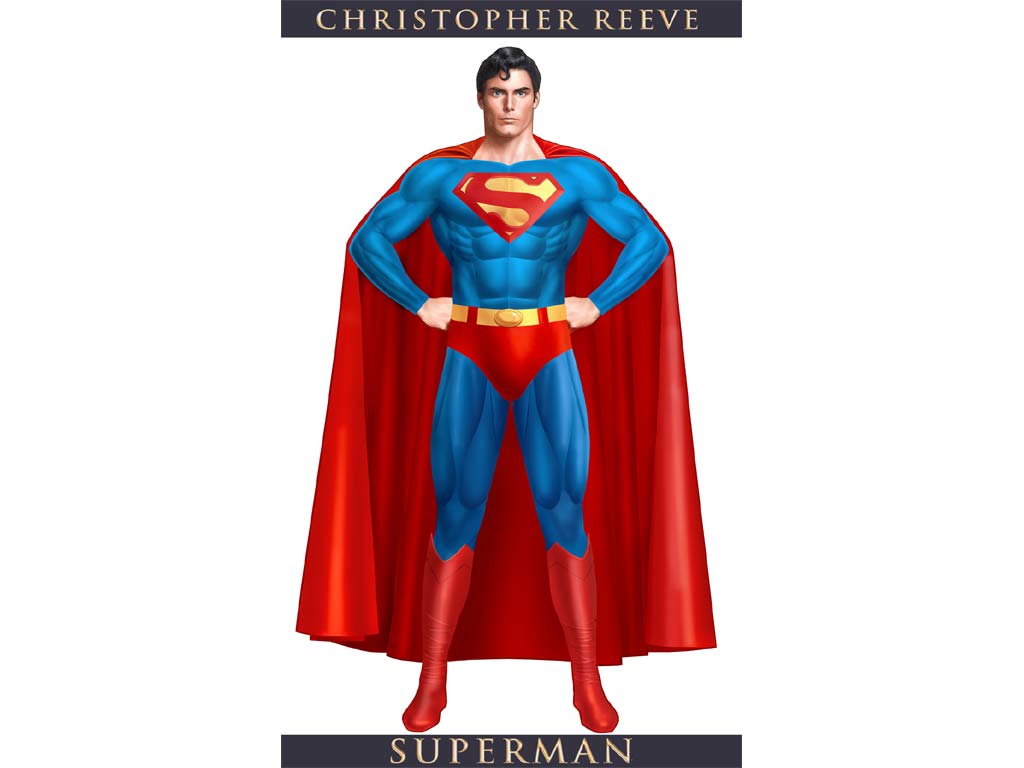The image features a highly detailed, brightly colored depiction of Superman, unmistakably portrayed by Christopher Reeve. Set against a completely white background, the image prominently includes black bars at the top and bottom. The top bar reads "Christopher Reeve," and the bottom bar reads "Superman" in bold block lettering. Reeve, dressed in the traditional Superman attire—a blue spandex suit with red 'underwear' on the outside, red boots, and a bright red cape—strikes an iconic stance. His muscular physique is meticulously defined, from his legs and stomach to his arms. He sports a signature 'S' emblem, encased in a diamond shape, on his chest. His hair has a distinctive curl on the forehead, and he wears a serious, solemn expression while looking directly at the viewer. The image, possibly a stylized movie poster, captures the essence of the classic superhero character, emphasizing Reeve's iconic portrayal.